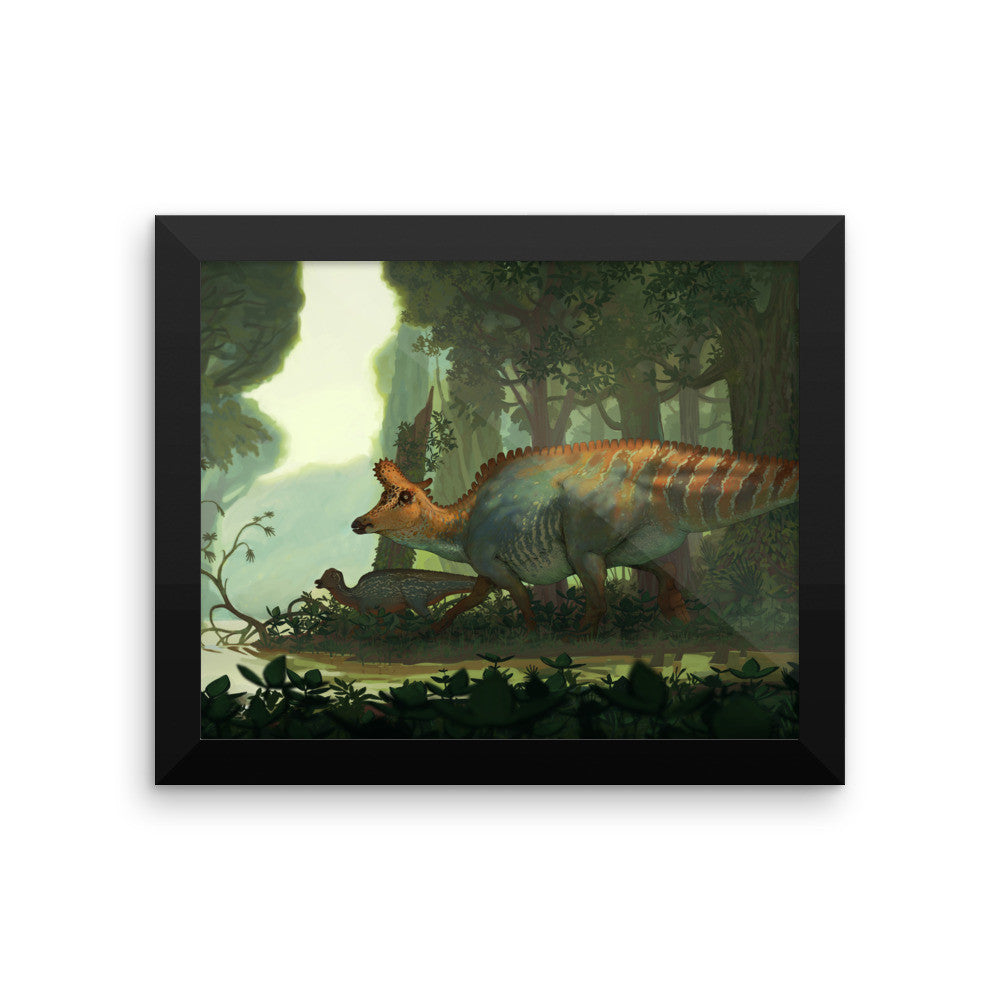This is an image of a painting displayed inside a rectangular black frame, set against a white background suggestive of a promotional product image. The painting captures two lizard-like dinosaurs standing beside a brown river in a lush forest. Each dinosaur features a long, horse-like snout with a crest on its forehead, black eyes, and orange-colored heads that contrast with their blue and white underbellies. Their backs are adorned with orange, red, and white stripes leading to their tails. They also possess spikes running from the head down to the tail. The scene includes a variety of green vegetation, including grass and small plants, with tall brown trees topped with green leaves surrounding the dinosaurs. The larger dinosaur looks protectively at a smaller one, possibly a mother and its baby. Dark gray clouds loom in the background, adding a sense of impending weather to the serene forest setting.